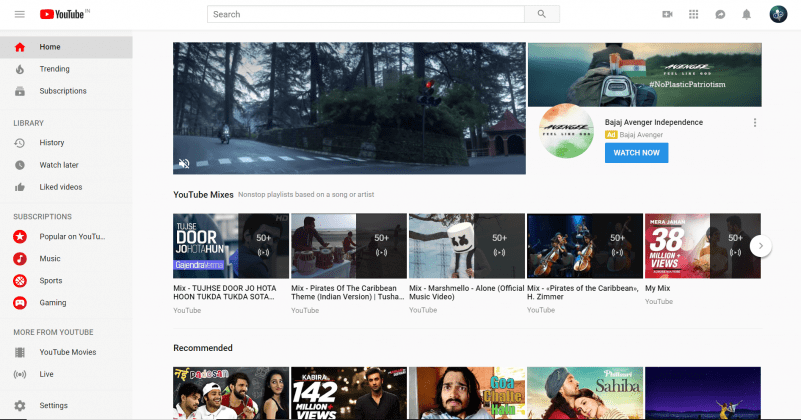The image depicts a YouTube interface, rich in details and icons, commonly seen on a computer screen.

On the far left, there is a vertical stack of three horizontal lines, commonly known as the hamburger menu icon. Next to it is the recognizable YouTube logo. Moving right, there is a horizontally outlined grey rectangle labeled "search" with a magnifying glass icon at its far right, serving as the search bar. Adjacent to the search bar, there's an indiscernible grey icon, followed by a grid of grey dots forming a square, typically indicating the apps menu. 

Next, there's a grey circle with a small white segment inside, and a grey bell icon, symbolizing notifications. Towards the end of the upper menu, there's a bluish circle with some white in it, likely representing a user profile or avatar.

Beneath the YouTube logo on the left, there's a horizontal line stretching across the screen. Below this line, there are several interactive menu items. The first one is a grey rectangle with a red house icon accompanied by the label "Home." Underneath, there is a lighter grey rectangle featuring an indistinguishable symbol and text. 

Following this are two more similar items with icons and labels that aren't clearly visible. The next section is labeled "Library," which contains three icon-item pairs. Below "Library," there is a "Subscriptions" section highlighted in red with four icons and accompanying grey text labels.

Another section titled "More from YouTube" appears in grey text, followed by more icons with illegible labels, which might include common features like "YouTube Music" and "YouTube Kids." There's also a gear-shaped icon indicating settings.

To the right, the central portion of the screen appears to show video recommendations or thumbnails. One image resembles a street with a house, another might depict someone on a motorcycle, though both are somewhat unclear. Below this, there is a colorful circular icon and a blue rectangle labeled "Watch Now," likely inviting the user to view a video. Further down are additional smaller images and labels, difficult to discern, suggesting more video recommendations or categories.

Overall, the interface is a standard representation of a YouTube homepage, brimming with navigational elements, icons, and thumbnail previews.